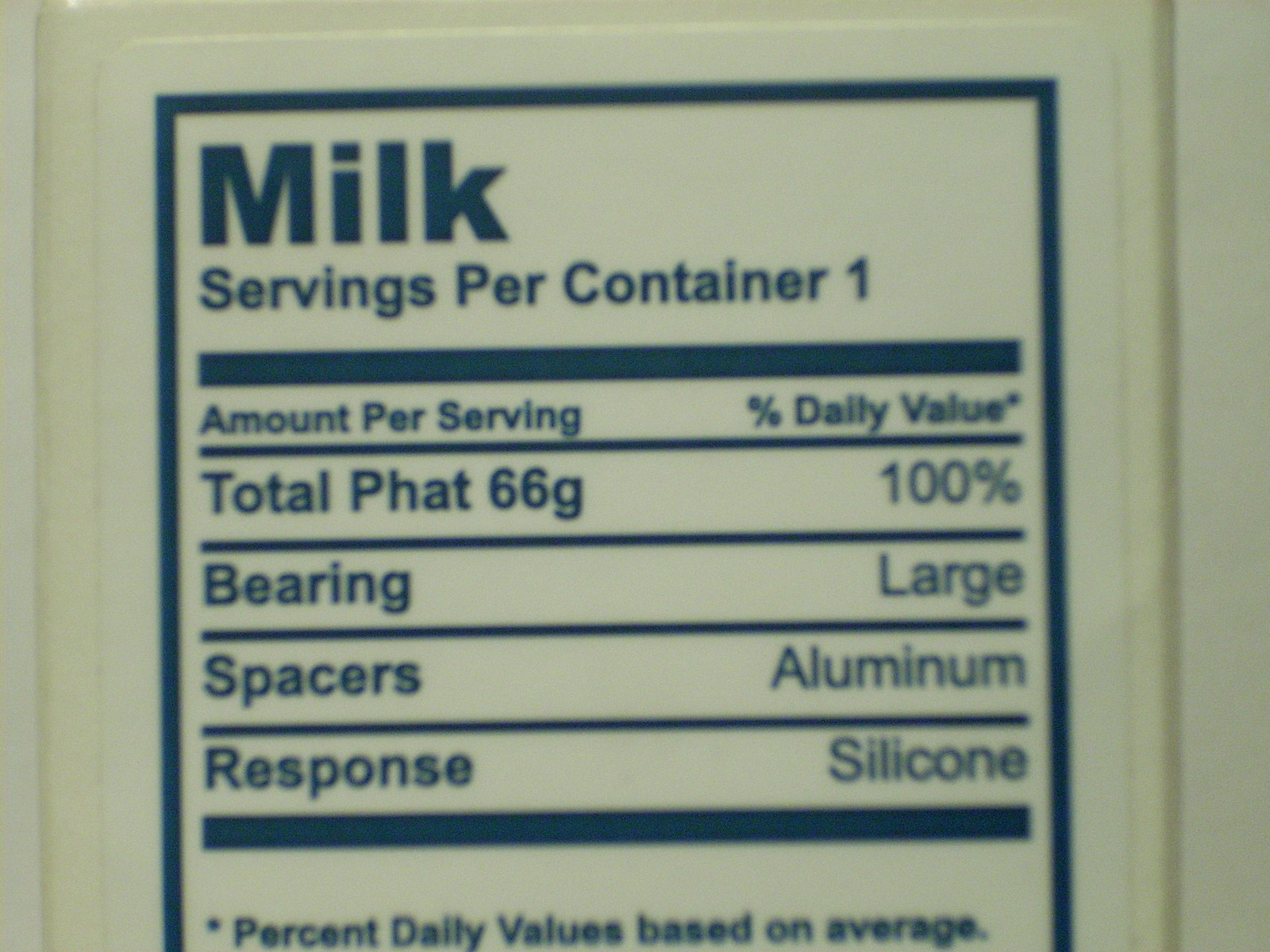This close-up photo showcases a heavily customized label on a milk carton. The label is a crisp white with dark blue printing and features a distinct blue trim. The image does not capture the full label but provides a generous amount of detail. At the top, "Milk" is displayed prominently in bold text with a capital "M" and lowercase "ilk." Directly beneath, it states "servings per container: one," followed by a thick horizontal line dividing the sections.

The next section is standard for nutritional labels, listing "Amount per serving" and "Percent Daily Value," denoted with an asterisk. The peculiar customizations start here. It lists "Total Fat," but spells fat as "P-H-A-T," assigning it a value of 66 grams and a daily value of 100%. Below this, unconventional categories appear, including "Bearing" with the daily value listed as "large," "Spacers" showing "aluminium," and "Response" noted as "silicone." 

Each section is separated by lines for clarity. At the bottom, nearly cut off in the image, an asterisk explains that the "Percent daily values based on average." The overall layout and specifics suggest this label is a playful or promotional alteration rather than a standard nutritional guide.